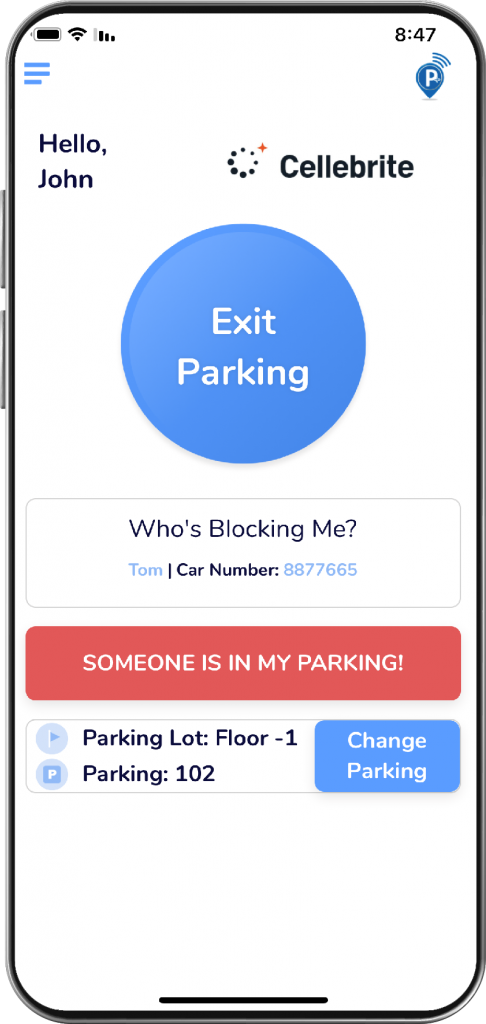This digitally created image mimics a mobile phone screen, showcasing a mobile application designed for managing parking situations. The edges of a smartphone frame the screen, highlighting its interface.

At the top of the screen, black icons display the battery life, WiFi connection, network signal, and the current time, reinforcing the mobile interface theme. On the top left, three blue vertical lines suggest a dropdown menu option, while the top right corner features a blue GPS pin icon with a 'P', denoting parking.

The main content area greets the user with "Hello John" and prominently displays a blue circular button labeled "Exit Parking". Below this, a notification box reads 'Who's blocking me?' followed by the details 'Tom, car number 8877665'. Adjacent to this, a red rectangular button offers the user an option to report that "Someone is in my parking". At the bottom of the screen, there is an option to "Change Parking", along with the designation of the specific parking lot number.

Overall, the image represents the user interface of a parking management app, providing various functionalities to monitor and resolve parking-related issues.